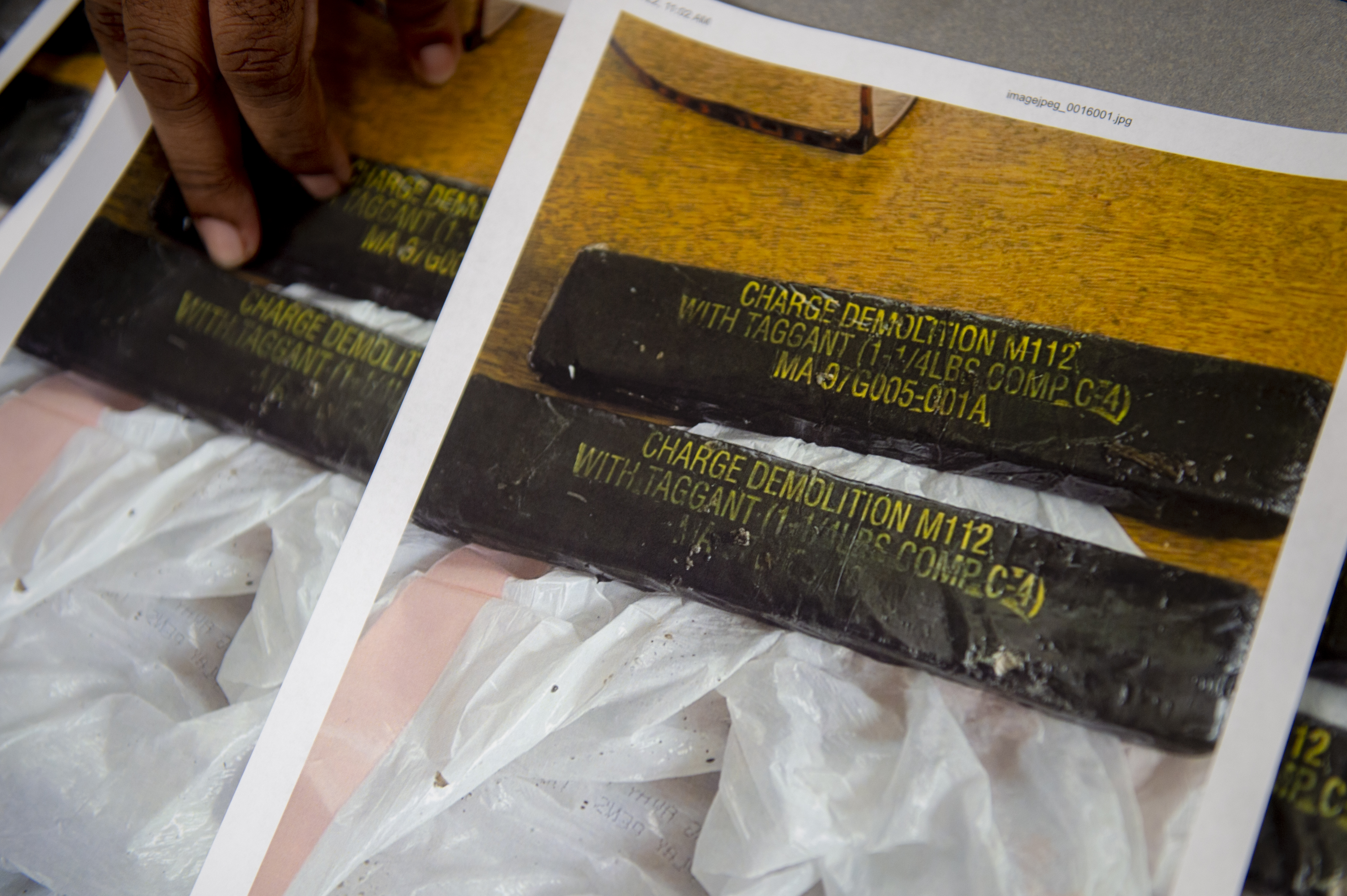In this detailed photograph, a stack of eight and a half by eleven-inch papers lies on a brown wooden surface, each sheet showcasing identical full-color images. The images prominently feature two black rectangular objects, likely sticks of C4 explosives, marked with yellow text that reads, "Charge Demolition M112 with Taggant, 1 1/4 pounds Comp C4,” along with additional details such as "MA97G005-001A." One of the objects has some text partially rubbed off. Both objects are placed on a white trash bag. In the top left corner of the uppermost paper, a pair of eyeglasses rests. Notably, the top paper bears a small black text in the upper white margin, which reads "imageJPEG_0016001.jpg," indicative of the file name. A hand, with visible fingers but not fully in view, appears on the left side of the top paper, suggesting someone is examining the documents. The overall setup seems meticulous and investigative, as if related to a crime scene or forensic analysis.